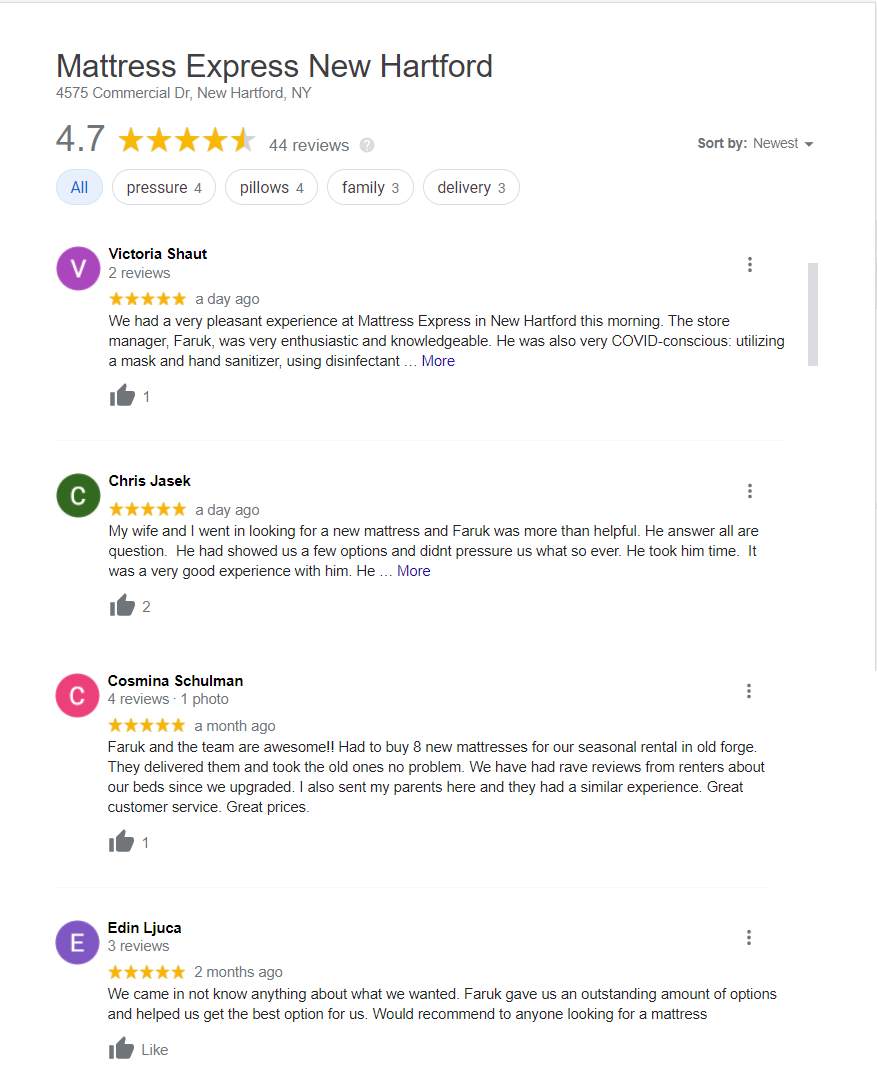Image Caption: The image showcases the top section of the Mattress Express website for the New Hartford, New York location, situated at 4575 Commercial Dr. The store boasts an impressive 4.7-star rating based on 44 reviews. The customer highlighted in the review, Victoria Shaw, gave the store a glowing five-star rating just a day ago.

In her review, Victoria mentioned their positive experience at Mattress Express that morning. She praised the store manager, Farrakh, for being very enthusiastic, knowledgeable, and COVID-conscious. Another review from Chris Jessicks emphasized that he and his wife received exceptional service from Farrakh and the team. They were looking for a new mattress and appreciated the helpful guidance provided without any pressure. The store even facilitated a seamless delivery for their seasonal rental, leading to numerous compliments about the upgraded beds. Chris also recommended the store to his parents, who enjoyed a similar excellent customer service experience at great prices.